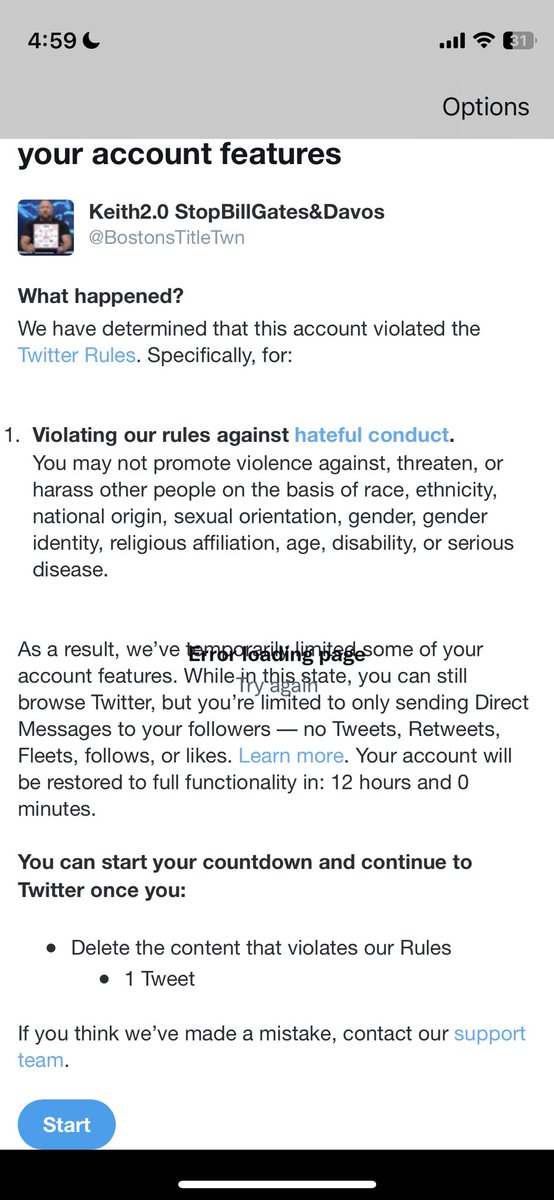The image is a vertically rectangular screenshot from a website, likely Twitter. The screen's top portion features a light gray horizontal banner displaying the time, 4:59, in the upper left corner, and icons for signal strength, Wi-Fi, and battery (which shows 31% remaining) in the upper right corner.

Below the banner, a menu options bar is partially visible, suggesting the page has been slightly scrolled down. The first visible line reads "Your Account Features." Directly beneath this, there is a user avatar followed by the name "Keith 2.0" and the phrases "Stop Bill Gates" and "Davos."

Further down, there's a notification from Twitter with the heading "What happened?" The notification states that this account violated Twitter rules specifically for "hateful conduct." The detailed explanation outlines that Twitter does not allow users to promote violence, threaten, or harass others based on race, ethnicity, national origin, sexual orientation, gender, gender identity, religious affiliation, age, disability, or serious disease.

The message continues, explaining the consequences and next steps. It instructs the user to "start your countdown and continue to Twitter once you delete the content that violates our rules," which includes one offending tweet. The notification concludes with an option to contact Twitter's support team if the user believes a mistake was made.